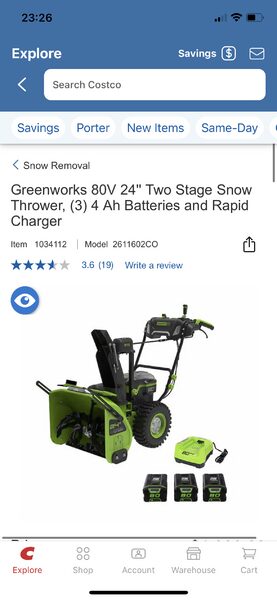A detailed screenshot of the Costco website featuring the header in a dark blue color. The header displays the word "Explore" on the top left, with icons for savings and mail on the top right, positioned just above the search bar. Below the search bar, there is a stripe in a very light blue shade with four tags labeled "Savings," "Order," "New Items," and "Same Day."

Below this stripe is the product page for a Greenworks 80V 24-inch Two-Stage Snow Thrower, complete with four AH batteries and a rapid charger. The item number for this product is 1034112, and the model number is 2611602C0. The product has received a rating of 3.6 stars from 19 reviews.

The snow thrower is illustrated with two wheels and a seat for the operator, which is not covered by any material. The main body of the snow thrower is green. Included in the image are the three four AH batteries and the charger.

At the footer of the website, the red Costco logo is visible with the text "Explore." To the right of the logo, there are navigation options labeled "Shop," "Account," "Warehouse," and "Cart."